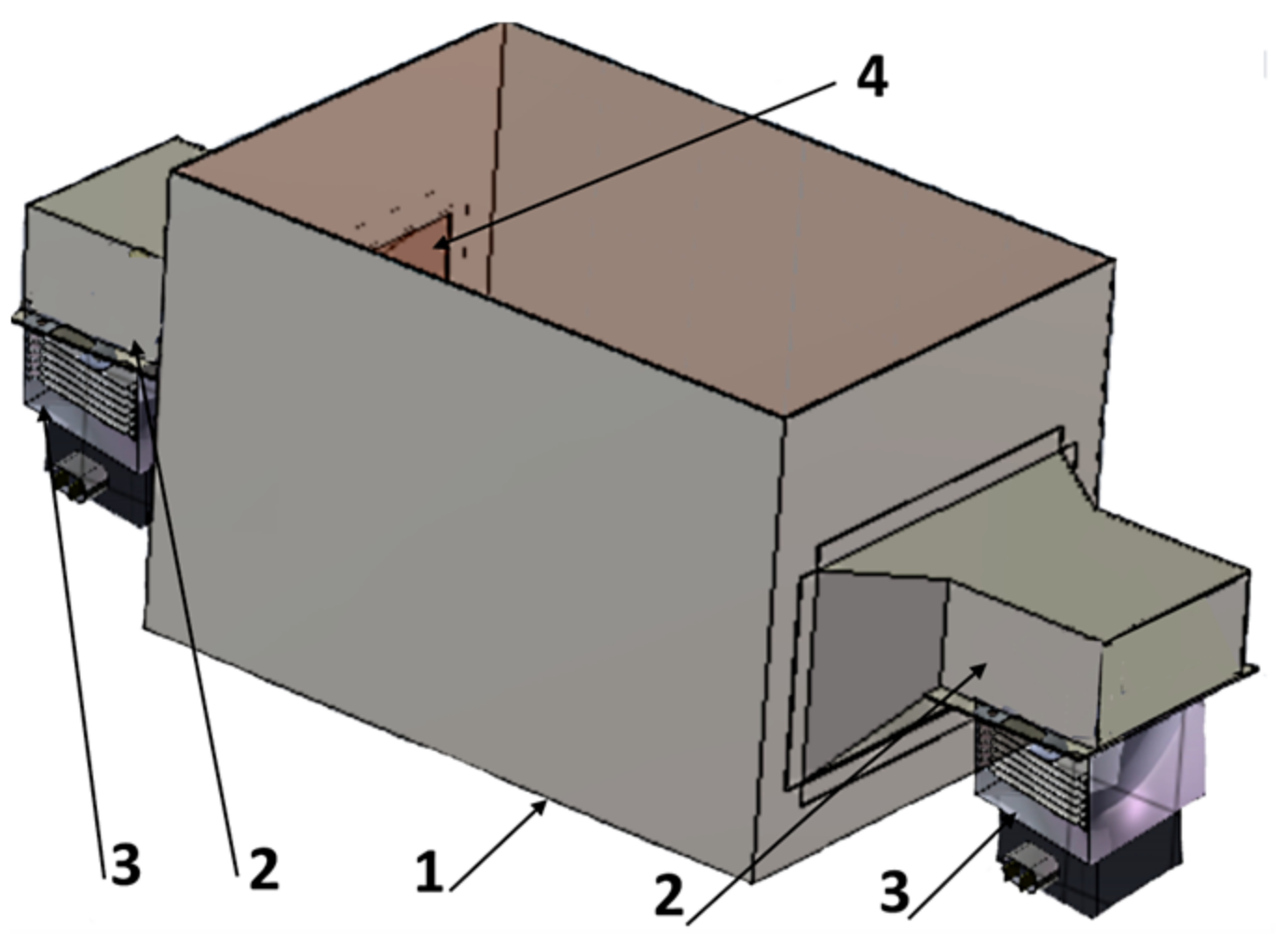The image is a detailed diagram depicting the self-installation process of a ventilation system, characterized by a central rectangular box with no openings on the short wall ends. The box is predominantly gray and resembles a room or an air conditioner. The diagram features four numbered components. Number one indicates the box itself, while number two is associated with an extending component on either end of the box. Number three is identified as the main part of this extension. Number four points to the interior of one of the short wall ends. The colors utilized in the diagram include gray, brown, lavender, and black, and the graphics are labeled without text, relying on numbers to indicate various parts. The numbers help guide the installation by showing where each of the four items should be placed, with specific placements such as near the bottom and in the interior sections. The components mentioned include a light spectrophotometer reader and its parts, which may use light to scan items within the system. Despite its detailed representation, the overall function of the box remains ambiguous, suggesting it could be a multifunctional unit involving both ventilation and light spectrometry.